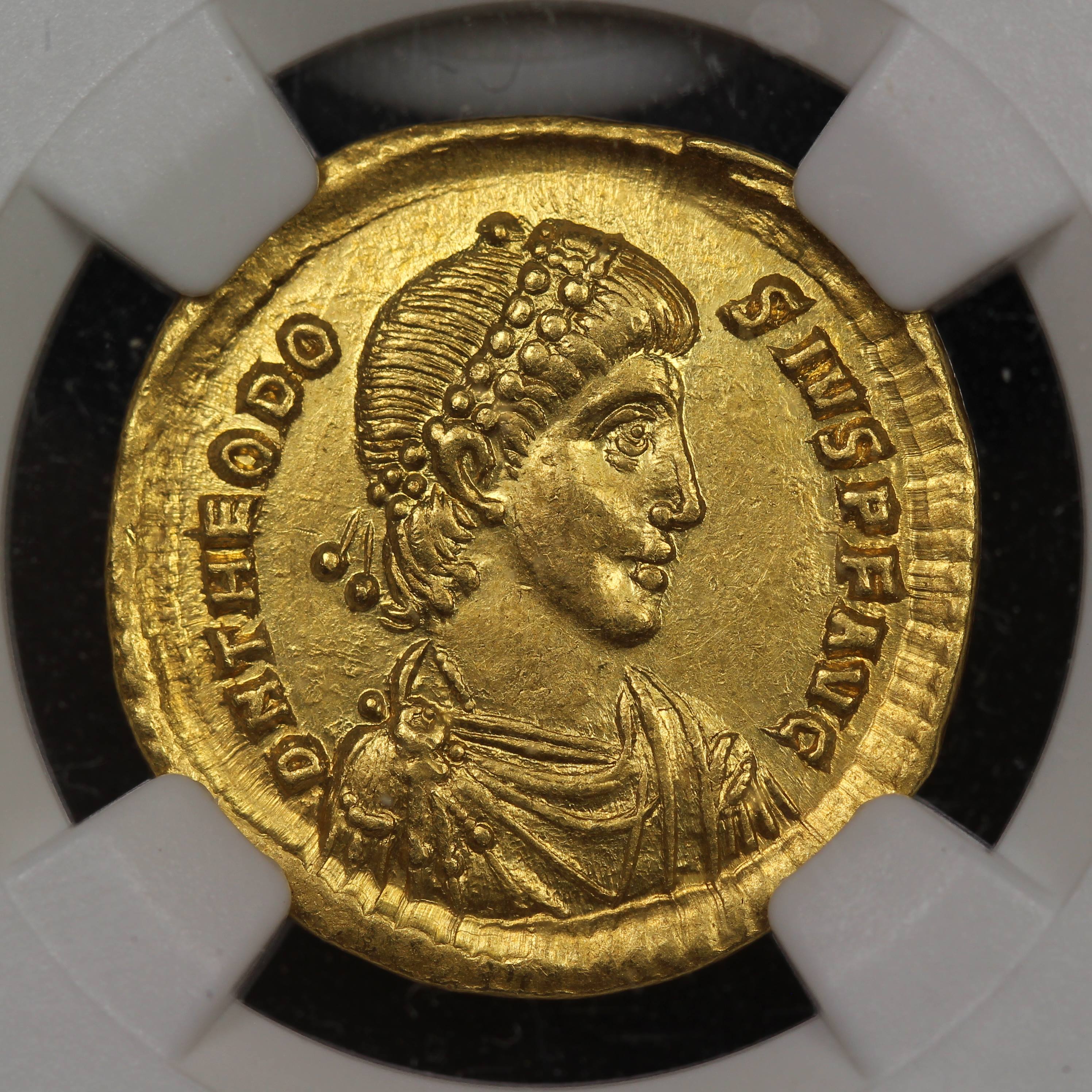This photograph showcases a detailed, gold coin featuring the likeness of Julius Caesar adorned with a wreath around his head. The coin, which lacks a visible date, is set against the backdrop of a protective black circle and is secured in place by a specialized container with four prongs, positioned at the top right, top left, bottom left, and bottom right. The intricate Latin inscription around the coin's edge, though partially captured due to clipping, suggests its historical significance. Centered within the image, the coin appears genuine and meticulously preserved, hinting at its placement in a special coin box or book designed to protect such valuable artifacts. The overall presentation, with the coin at the center and its protective casing adding a stark black and white contrast, accentuates its ancient Roman styling and esteemed status.